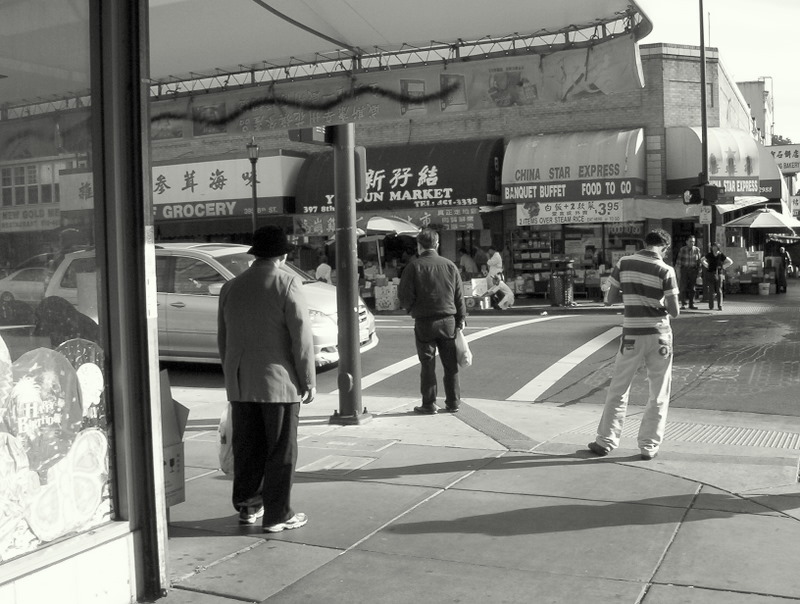This is a horizontal rectangular black and white photograph capturing a vibrant street corner in an Asian city. The image features text in both Asian characters and English. At the forefront, a man in white pants and a dark striped shirt holds his gaze downward, likely focused on his phone. To his left, three men, dressed in darker attire, stand by the crosswalk, possibly waiting for the traffic light to change. A storefront window adjacent to the crosswalk displays images, potentially balloons with "Happy Birthday" messages. Vehicles are parked and moving in the background, contributing to the bustling street scene.

On the opposite side of the street, a market, identifiable by prominent English signage reading "China Store Express" and "banquet buffet, food to go," advertises a meal for $3.95. Multiple people can be seen strolling past, adding to the busy urban atmosphere. The scene is anchored by the daily routines of the city's inhabitants, offering a snapshot of life at this particular street corner.